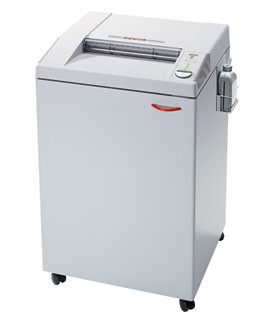Set against a white background, the image depicts a sizable, off-white, rectangular office paper shredder, notable for its old-school, bulky design. A red curved handle is attached to the top right corner of the front, likely used for accessing the shredded paper compartment. The top of the shredder features an angled cutaway revealing the blades for shredding paper, accompanied by text and a prominent red word in the center. To the right of the paper inlet is a control knob adorned with red and black lettering. The shredder also includes buttons in various colors: white, green, and a yellow dot.

On the right side of the machine, near the top back corner, there is a small caged compartment holding a silver bottle, possibly containing lubricant. The shredder sits on black roller wheels, which can turn easily in different directions, visible beneath the front left, right, and far right sides of the device. Overall, its size and features suggest it is designed for communal use in an office environment.